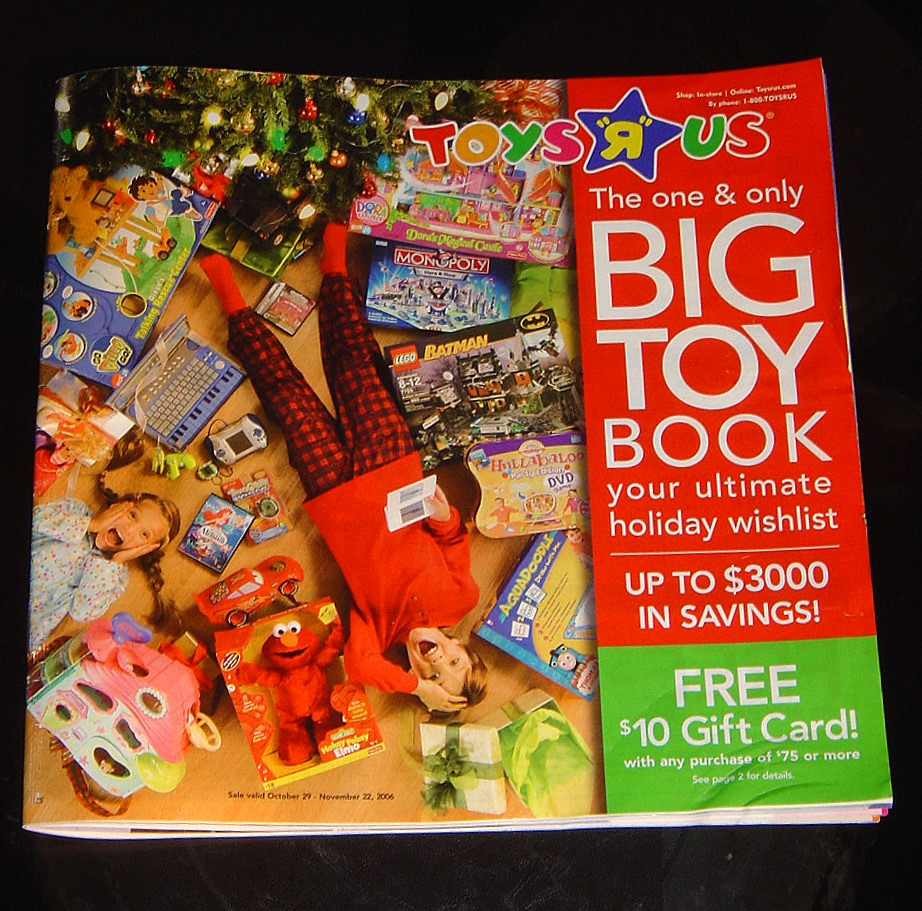This image features the cover of a Toys R Us catalog sprawled across a black surface. Dominating most of the image, the catalog is shown with only slivers of the surface visible around its edges. In the top right corner, the iconic Toys R Us logo is prominently displayed. A vertical red line divides the catalog, with approximately three-quarters of the cover to the left and one-quarter to the right.

On the left-hand side, the scene is set for Christmas with a festive tree adorning the upper section. Beneath the tree lies an amazed redheaded boy clad in red socks, red and black checkered pajama pants, and a red shirt. His feet extend under the tree at the top of the image, while his head points towards the bottom. He holds a Nintendo DS in one hand, with the other resting on his forehead in awe. Next to him, a little girl with pigtails exhibits similar amazement, her mouth wide open and her hands on her cheeks. She, too, is in pajamas.

The children are surrounded by an assortment of toys and gifts, including a Tickle Me Elmo doll, Batman Legos, a Monopoly board game, electronic games, and an array of open Christmas presents. The right side of the catalog features the text "The one and only Big Toy Book" in bold white letters, along with "Your Ultimate Holiday Wish List" and "Up to $3,000 in savings". At the bottom right corner, a green box announces a "Free $10 Gift Card with any purchase of $75 or more". Additionally, the bottom of the catalog indicates the sale dates as valid from October 29th to November 22nd, 2006, suggesting the catalog is from that year.